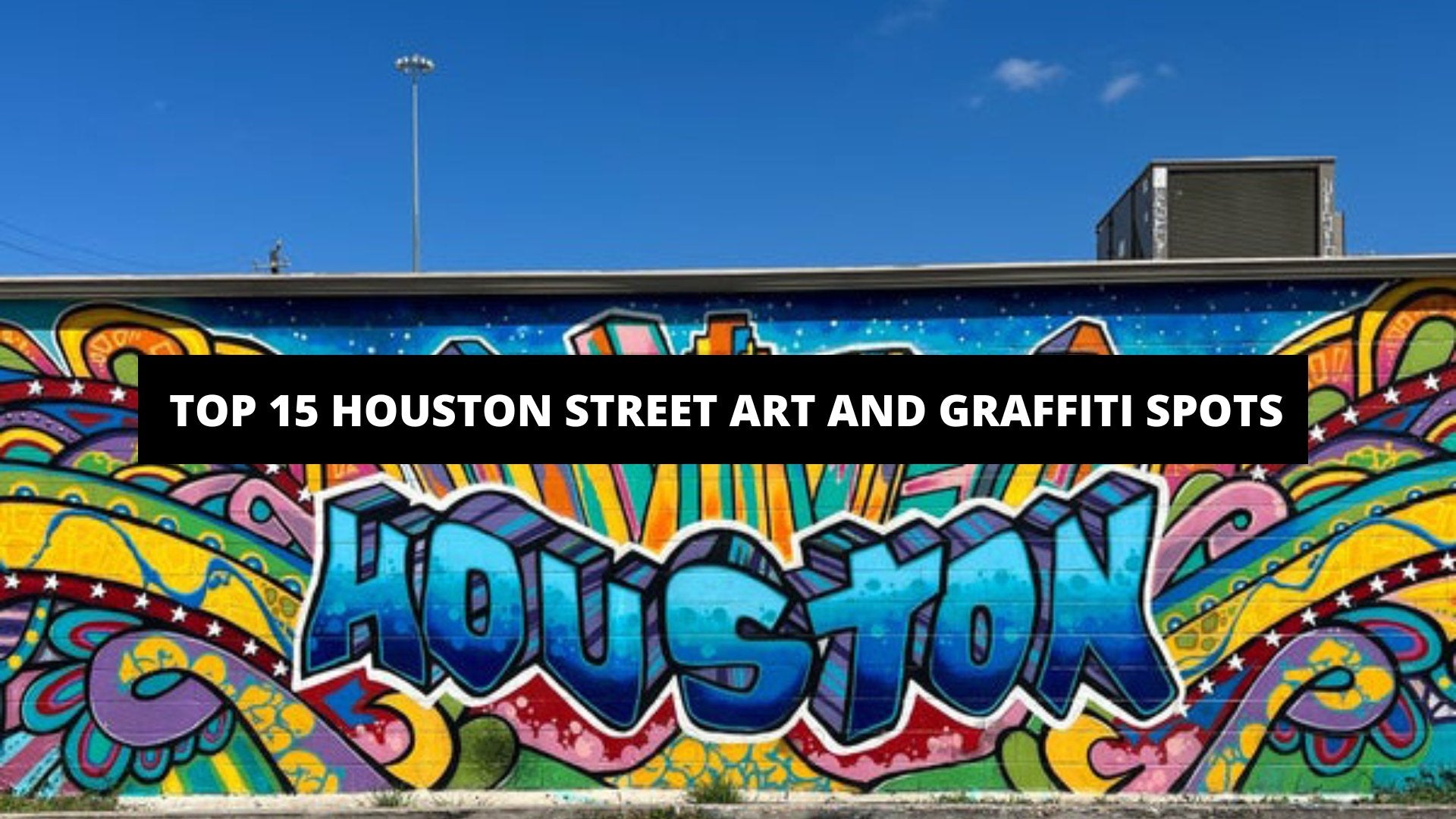The image features a vibrant piece of street art painted on the side of a building, set against a bright blue sky with wispy white clouds. The main focal point is the word "Houston" displayed in large, blue, block letters with an ombre effect, transitioning from a lighter shade at the top to a darker one at the bottom. The artwork is adorned with a dynamic array of colorful squiggly lines and graphics in various hues such as yellow, green, blue, orange, and light purple. Superimposed on the graffiti is a black rectangular banner with white text that reads, "Top 15 Houston Street Art and Graffiti Spots." The building's roof and an air conditioner are visible, adding to the urban setting. This image appears to serve as an advertisement, likely for a blog or article detailing Houston's notable street art locations.